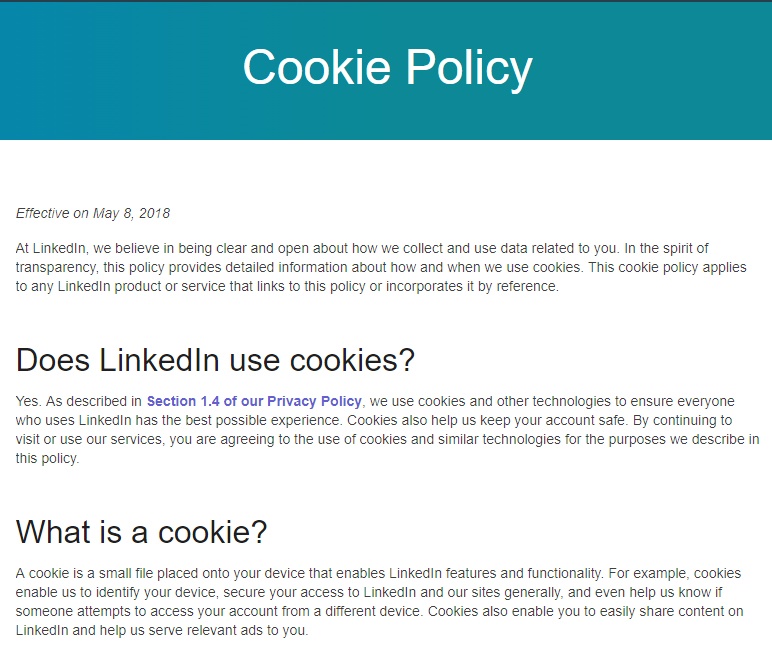This image features a screenshot of a LinkedIn cookie policy displayed in a visually distinct blue box. The heading "Cookie Policy" is prominently displayed at the top in white font with capitalized letters "C" and "P". Directly underneath, the text reads "Effective on May 8th, 2018".

The main body of the policy begins with a statement emphasizing LinkedIn's commitment to transparency regarding data collection and usage. The policy elaborates that it provides comprehensive details about LinkedIn's use of cookies, which is applicable to any LinkedIn product or service referencing this policy.

Following the introduction are sections in a Q&A format. The first question, "Does LinkedIn use cookies?" appears in black lettering and is affirmatively answered with a direction to section 1.4 of LinkedIn’s privacy policy for further details.

The next question, "What is a cookie?" is also answered in detail. It describes a cookie as a small file placed on your device that enables various LinkedIn features and functionalities. Examples include device identification, securing access to LinkedIn, and detecting unauthorized access attempts.

This screenshot provides a clear and detailed explanation of LinkedIn's cookie usage policies and their application, adhering to a transparent user engagement approach.